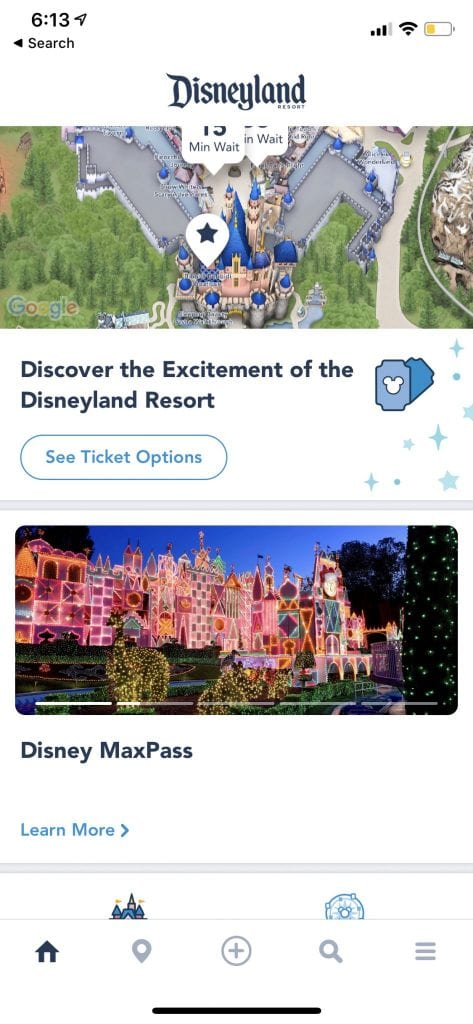This screenshot from a cell phone features multiple elements associated with Disneyland displayed on a vibrant screen interface. At the top portion, the word "search" is prominently positioned on the left-hand side in smaller font, accompanied by a back arrow icon directly above it.

Beneath this, the first section is dedicated to Disneyland and is center-justified, with the word "Resort" neatly placed under the 'N' and 'D' in "Disneyland." The accompanying image within this section is a cartoony aerial view of the Disneyland castle, presented as a Google map picture. A speech bubble within this map image indicates the castle and a 15-minute wait time, enhancing the interactive appeal.

Following this, the screen prompts users to "Discover the excitement of the Disneyland Resort," enticing further engagement. 

Below this is the section titled "Disney MaxPass," distinguished by a scrolling bar of images related to Disneyland positioned above the title. The first image in this scrolling bar aligns slightly above the "Disney MaxPass" title, completing the visual journey through the various Disneyland-associated features. This detailed and vibrant layout guides users through the app's offerings seamlessly, emphasizing the excitement and utility of the Disneyland Resort and its attractions.